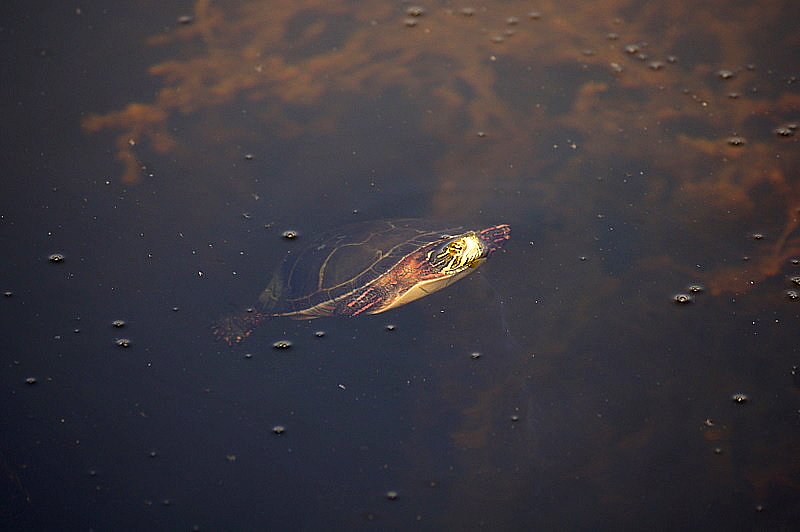The photograph is a horizontal-rectangular image, predominantly dark in tone, capturing a turtle in a large body of water. The scene, tinged with earthy hues, displays the turtle prominently in the center, its body partially submerged and its head poking out towards the surface. The turtle has a complex palette of colors, including shades of brown, dark brown, and sections of the shell and body exhibiting lighter browns, oranges, and hints of yellow. The water, tinted brown, adds to the overall dimness of the image. Overhead, the sky appears cloudy, subtly illuminated, contributing to the natural setting. The photograph is outdoor with the scene bathed in diffuse natural light, emphasizing the serene moment of the turtle in its aquatic environment. The image is void of any other animals, people, or objects, drawing complete attention to the turtle as it floats gracefully in the dark water.